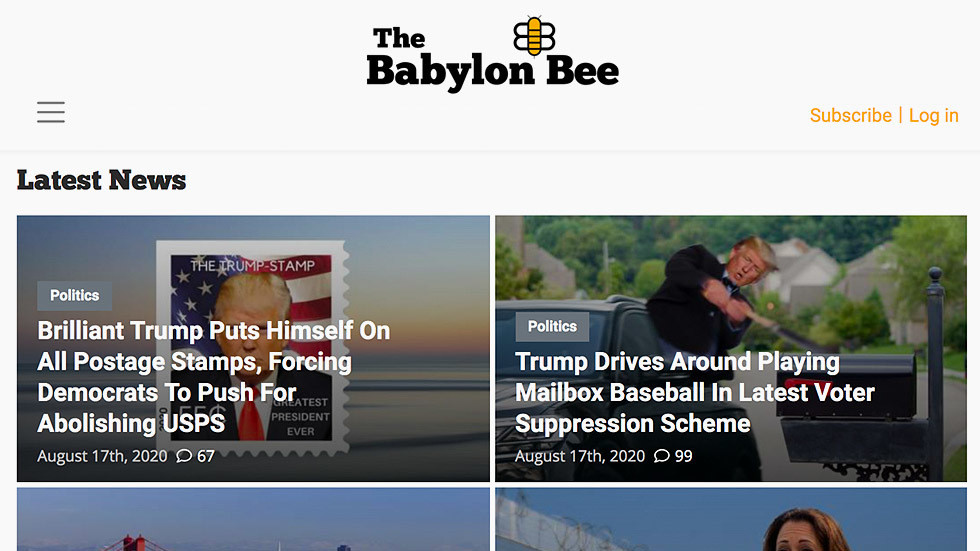This screenshot is from the right-wing satirical comedy news site, the Babylon Bee. The layout features a clean, minimalist design with a white background and a header at the top reading "The Babylon Bee" in black text, accompanied by their distinctive logo—a honey bee with two pairs of wings shaped like the letter "B." 

The main content displays partial previews of four articles, but only the top two are fully visible. 

The first article is titled "The Trump Stamp" and is accompanied by an image of former President Donald Trump depicted on a postage stamp, portrayed with an exaggeratedly orange complexion and set against an American flag backdrop. The subheadline humorously claims, "Brilliant Trump puts himself on all postage stamps forcing Democrats to push for abolishing the USPS."

The second article, positioned to the right, features a picture of Trump leaning out of a car and striking a mailbox with a baseball bat, captioned, "Trump drives around playing mailbox baseball in latest voter suppression scheme." Both articles were published on August 17, 2020.

Below these, only partial images and headlines of additional articles are visible, cut off at the bottom of the screenshot.